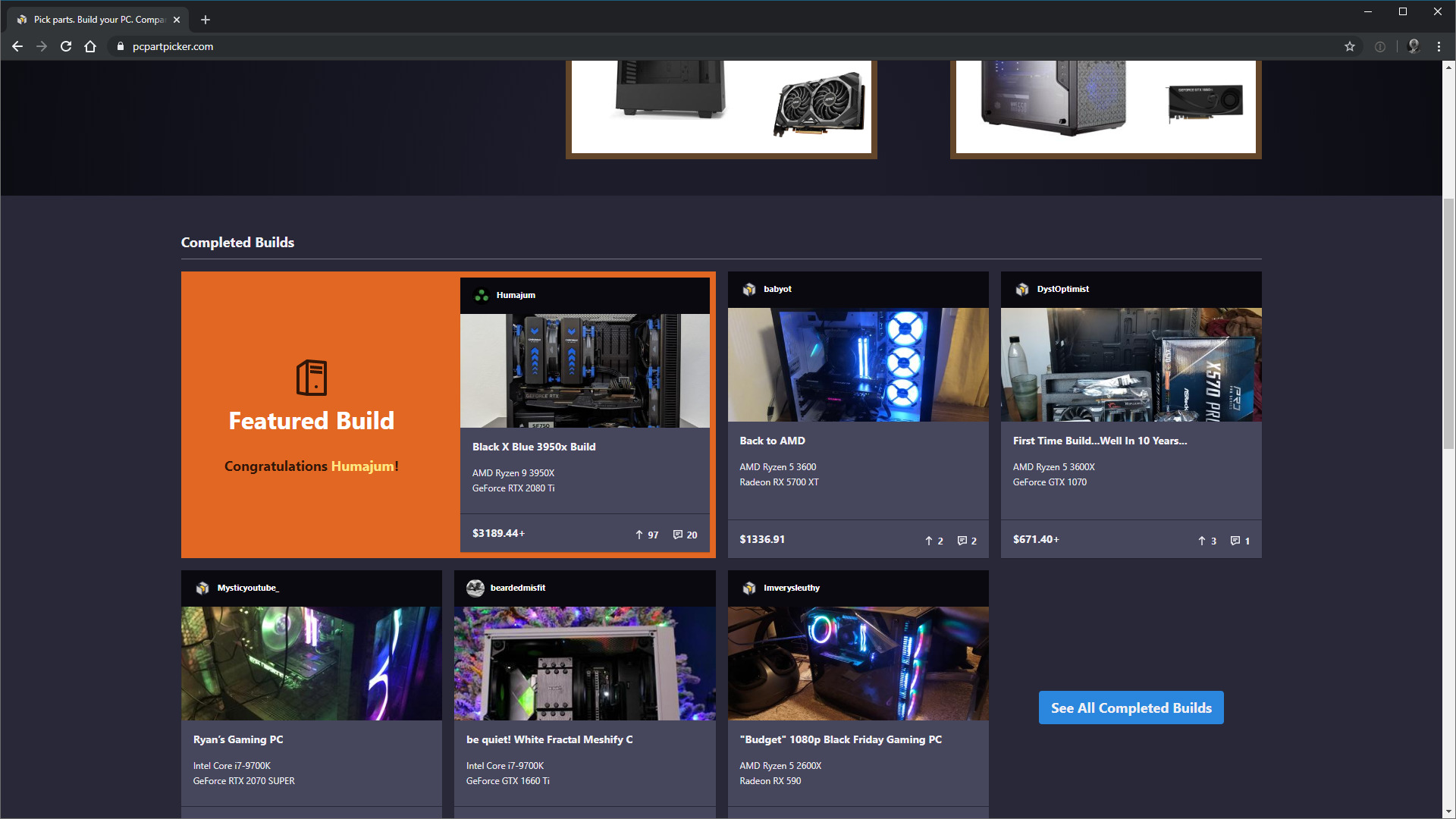The image is a screenshot from the website pcpartpicker.com, a platform used for selecting components for building custom PCs, with detailed information on pricing and availability. The main featured build highlighted in orange is a high-end setup by Hajime, named "Black Blue x3950x Build," which includes an AMD Ryzen 3950x CPU and a GeForce RTX 2080Ti GPU, priced at $3189.44. 

Another highlighted build, "Baby Op," also uses AMD components with a Ryzen 5 3600 CPU and a Radeon RX 5600 XT GPU, with a total cost of $1336.91. Additionally, there's a more budget-friendly option labeled as a first-time build in 10 years, featuring an AMD Ryzen 5 3600x CPU and a GeForce GTX 1070 GPU, priced at $671. The rest of the page showcases three other PC builds with varying prices and configurations, many of which feature RGB lighting, providing vibrant, customizable color displays. 

Overall, the website facilitates the process of assembling a PC by offering detailed component lists, images, and price breakdowns.